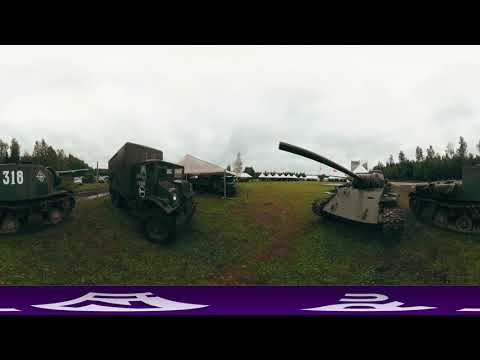In this image, we see a detailed military exercise or display set in an outdoor field during the middle of the day. The scene is bordered by a solid black band at both the top and bottom edges, and a purple banner featuring text in a foreign language runs across the screen. Central to the image is a flat, grassy field with patches of brown and green terrain. Positioned across the field are several military vehicles, including tanks and a half-track, occupying the entire center from left to right. 

On the left, a massive green metal object features the number 318. Next to it is a military truck’s head, and just behind are tan and white tents, suggesting a base camp. A prominent tank in the foreground faces forward, with its turret and gun barrel fully extended, while another tank behind it heads in the opposite direction. On the right side of the image, there are metal beige-gray objects including one with a large pipe protruding from the center and another green object with a belt around its base.

The background features additional tents with white tops, flanked by tree lines on either side, providing a natural enclosure to the setting. The sky above is predominantly white with hints of blue, emphasizing the daylight. The color palette includes hues of black, purple, green, brown, tan, gray, and white, painting a vivid picture of this military scene.